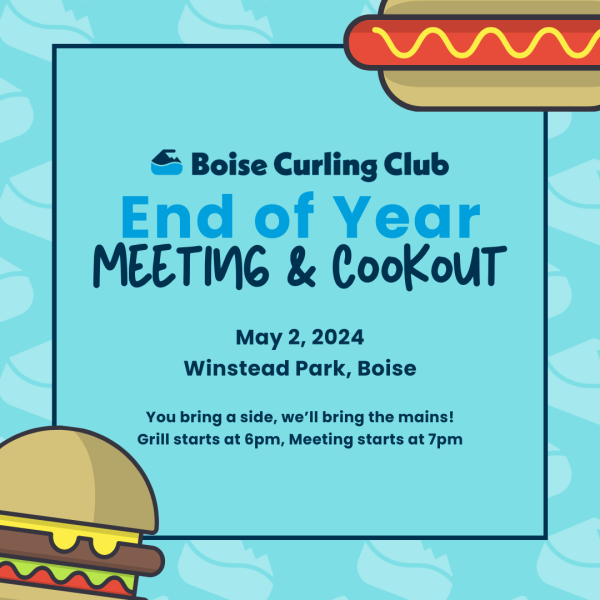The advertisement graphic for the Boise Curling Club's end-of-year meeting and cookout is predominantly blue, with a border featuring lighter blue designs, possibly leaves. The graphic is square in shape, approximately six inches by six inches. At the top right, there is an illustration of a hot dog with a brown bun and a red hot dog topped with a mustard stripe. In the bottom left, there is an image of a cheeseburger, complete with a brown bun, yellow cheese, brown patty, green lettuce, and red tomato. Central to the graphic is dark blue text that reads: "Boise Curling Club," followed by "end of year," and "meeting and cookout." Below this, it specifies the date and location: "May 2nd, 2024, Winstead Park, Boise." At the very bottom, the smallest text announces: "You bring a side, we'll bring the mains. Grill starts at 6pm, meeting starts at 7pm."